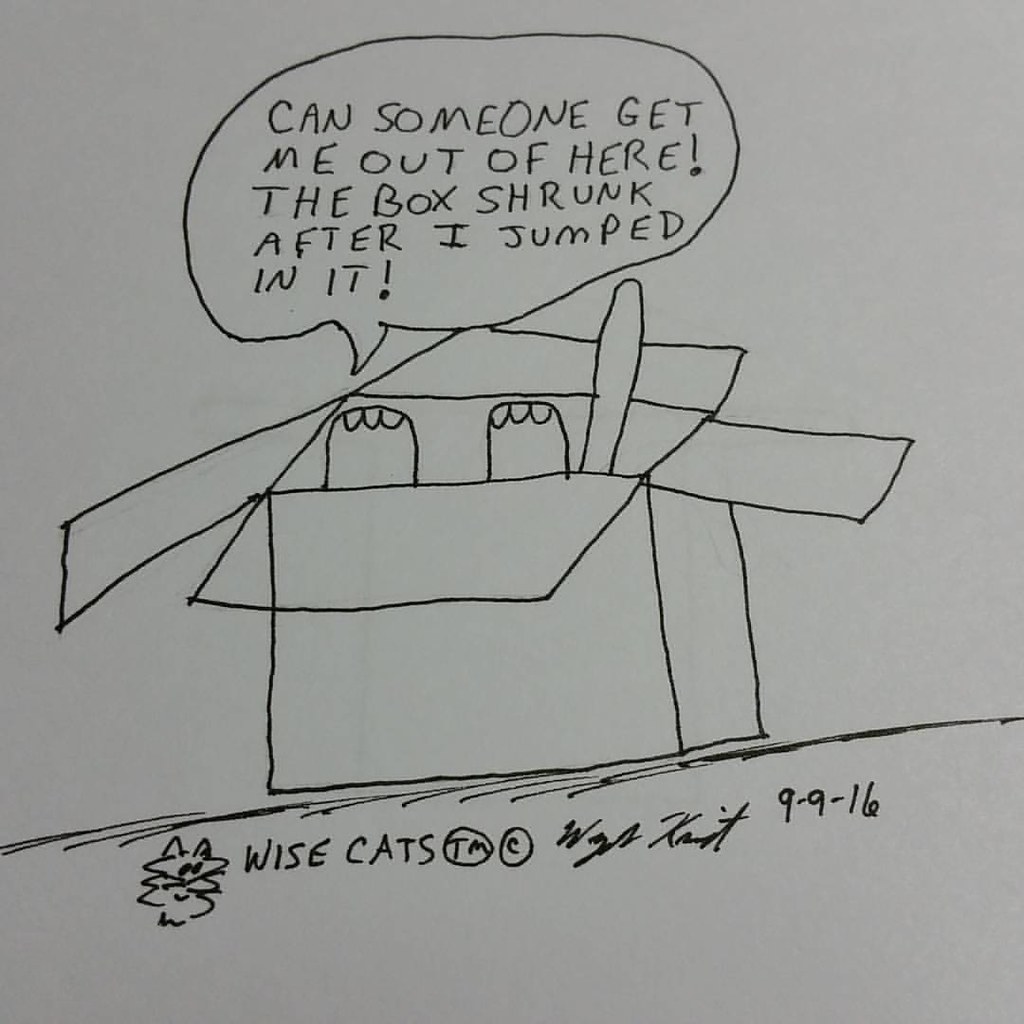The image is a hand-drawn sketch on a white piece of paper, created with thin black pen lines. The central focus is a rough drawing of a 3D cardboard box with all its flaps open, but the lines are not perfectly straight, adding a sketchy, spontaneous feel to the artwork. Inside the box, two animal-like feet and an arm are protruding, suggesting a creature is attempting to escape. Above the box, there’s a speech bubble in all capital letters stating, "CAN SOMEONE GET ME OUT OF HERE? THE BOX SHRUNK AFTER I JUMPED IN IT." Below the box, a scribbled line represents the floor, and near the bottom left is a rough, iconic drawing of a cat. The image includes the text "Wisecatz TM," along with a copyright symbol, a signature, and the date "9-9-16." The overall style is informal and gives the impression of a spontaneous, humorous doodle.